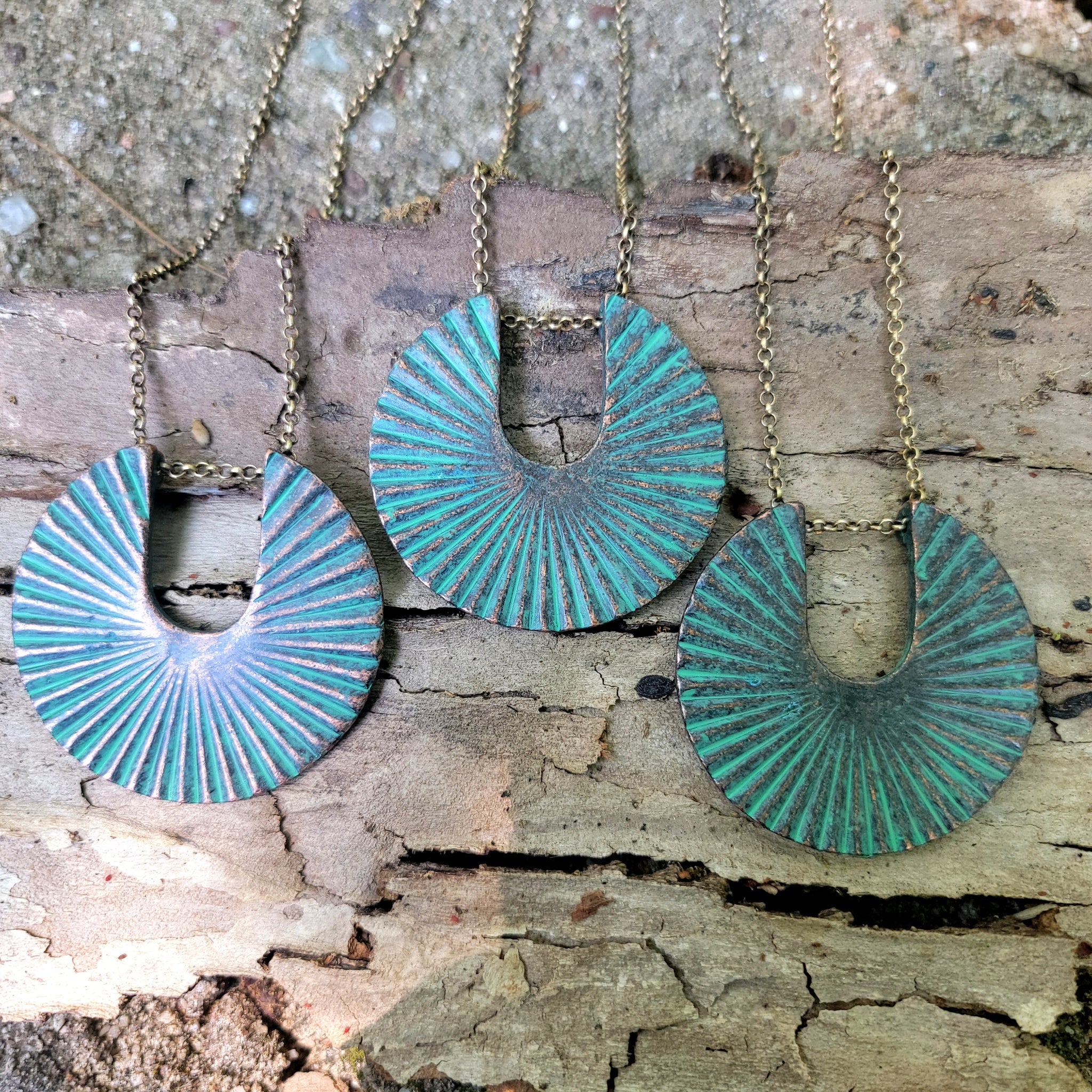This square, color photograph presents a detailed, zoomed-in view of three similar yet distinct brass-chained necklaces displayed artistically on a rustic, unvarnished piece of bark, likely from a hollow log. The pendants, shaped like nearly complete fans with a U-shaped cut out at the top for the chain, exhibit intricate designs reminiscent of oysters. They showcase a turquoise and metallic green hue, suggesting a blend of copper elements. One pendant on the far left stands out slightly more, reflecting light with a sunburst pattern in green, white, and touches of blue, while the other two pendants gravitate towards darker green and black tones. Bright colored cement accents at the top of the log add a modern, photorealistic aesthetic akin to listings seen on Etsy or small shop websites, creating an inviting, artisanal appeal.